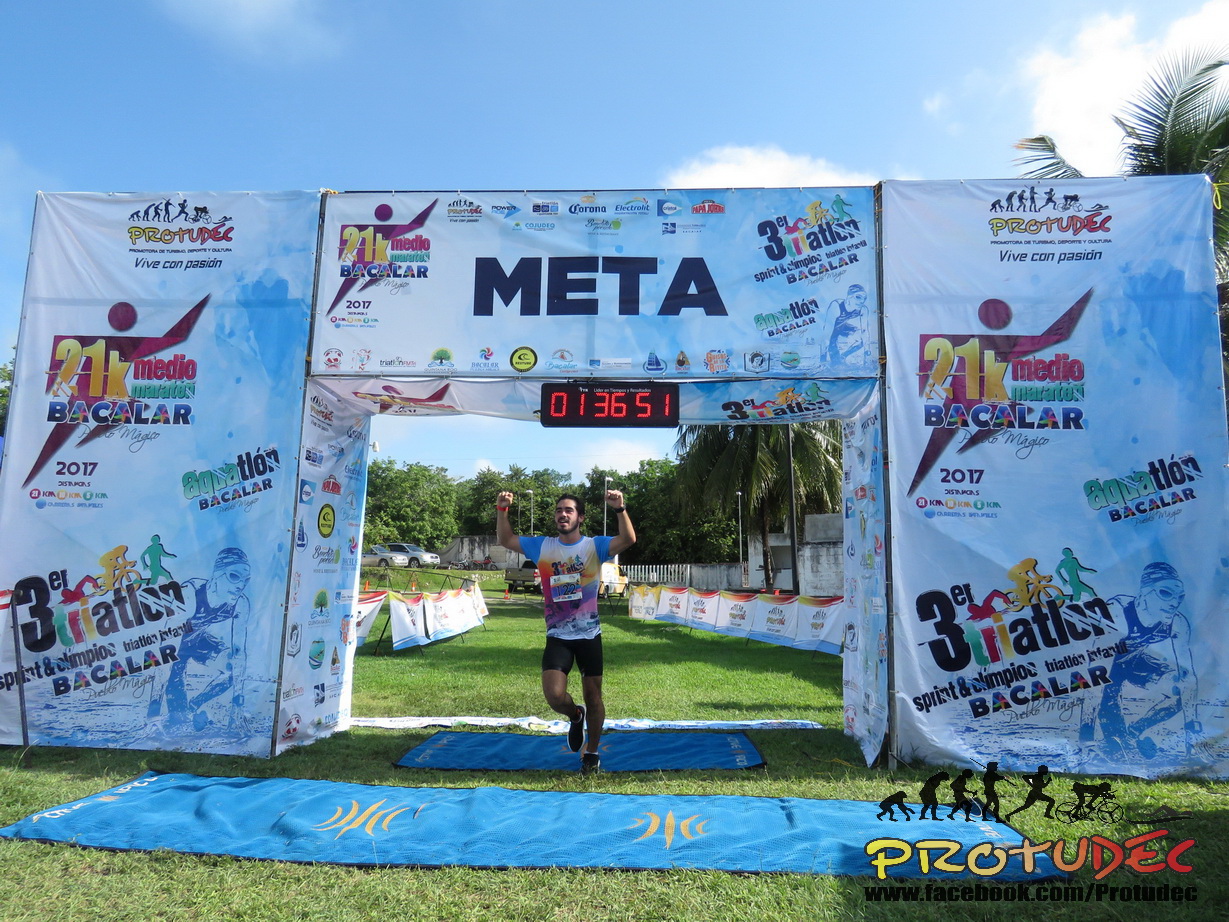The image captures a triumphant moment during a running competition, portraying a runner crossing the finish line under a makeshift arch made of steel tubing and banners. The arch prominently features the word "META" in bold, all caps, with various sponsor logos, including Bacalar and Protudec, displayed in primary colors like red, blue, yellow, and green. A digital clock above the runner shows the finishing time of 1:36:51. The runner, dressed in black shorts and a white shirt with blue trim, strikes a victorious pose with both fists raised. The scene is set against a grassy area with numerous palm trees, and the path is lined with white banners and covered with a blue mat. The setup and decorations suggest a professionally organized race, although no spectators are visible outside the arch.